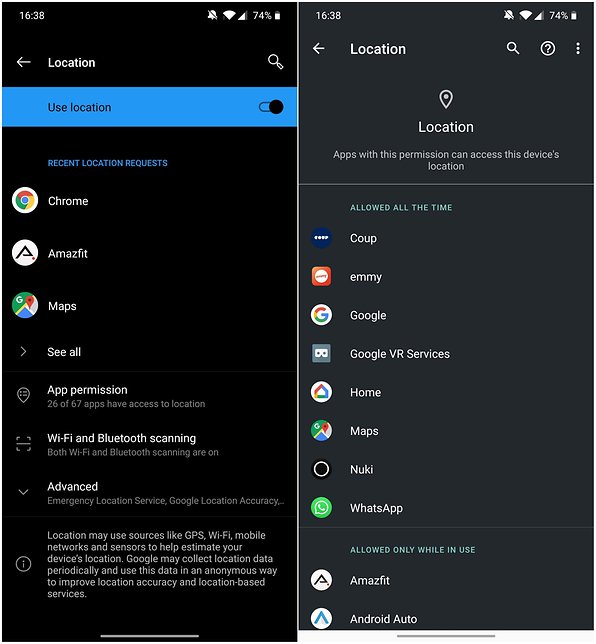The image features two side-by-side screenshots of the same cell phone taken at nighttime. Both screens display the time in military format, 16:38 (4:38 PM), and indicate a battery level of 74%. 

The screenshot on the left shows a darker interface with a deep black background. It highlights the "Use on location" settings, revealing that the location services are turned on. It lists recent location requests from apps such as Chrome, Amazon, Mi Fit, and Maps, with an option to view more. It also shows that Wi-Fi and Bluetooth scanning are enabled, and explains that location data may be collected periodically by Google to enhance accuracy and location-based services.

The screenshot on the right has a slightly lighter, dark charcoal background. It focuses on location permissions and displays a pinpoint icon indicating that location services are active. It lists the apps with location access, including those with "allowed all the time" permissions like Coop, Emmy, Google, Google VR Services, Home, Maps, Nuki, and WhatsApp. Additionally, it shows apps that are only allowed to access the location while in use, such as Amazon Fit and Android Auto.